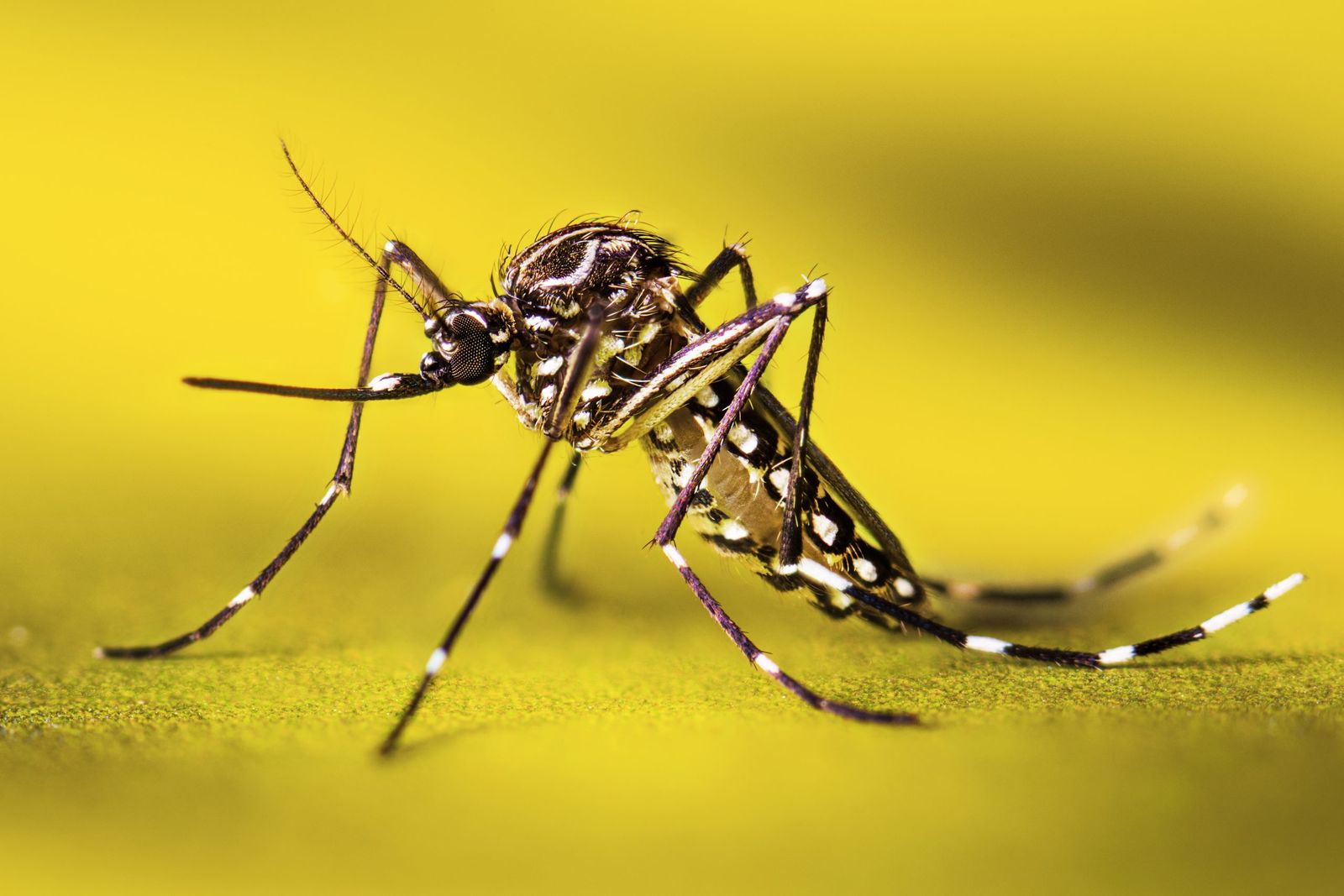This image is a very close-up shot of an insect, possibly a mosquito or cricket, showcasing intricate details. The insect is perched on a bright yellow surface, which makes the creature stand out starkly against the blurred yellow and brown background. Its elongated body is primarily brown, adorned with numerous white flecks. The antennae and the pointed stinger-like organ extend from its head, suggesting its predatory or defensive function. The insect's legs are incredibly long and thin, segmented with alternating bands of black and white, giving them a striking appearance. The legs, being black with white tips, resemble the pattern of a rattlesnake. The golden head and brown body with oval white spots bordered in black add to its distinguished look. Despite its common confusion with crickets or mosquitoes, the peculiar details of its anatomy, such as the segmented legs and the absence of wings, make this insect a captivating and somewhat enigmatic subject.